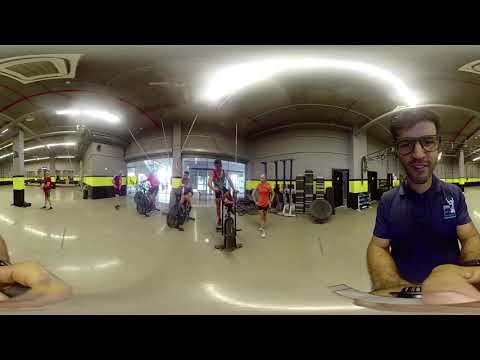The image portrays the interior of a gym with a distinct panoramic distortion. The gym itself is housed in a spacious, grey metal building accented by a yellow and black stripe at the lower third of the walls, and features large glass entryways and windows. The floor appears to be light-colored linoleum. In the foreground on the right, a young, bearded Caucasian man with big black glasses, dark hair, and a mustache, wearing a dark blue polo shirt, is captured—his proportions exaggerated due to the panoramic effect. His limbs and head seem disproportionately large, drawing attention to the distortion. The gym background shows several people engaged in various exercises: three individuals on exercise bikes in red and pink tops are near the left-center, a woman in an orangey-pink shirt performs split squats towards the center, and others are scattered, engaged in different activities. The space exudes an open, warehouse-like atmosphere, supported by numerous beams and an unobstructed layout, enhancing the sense of an expansive and active environment.